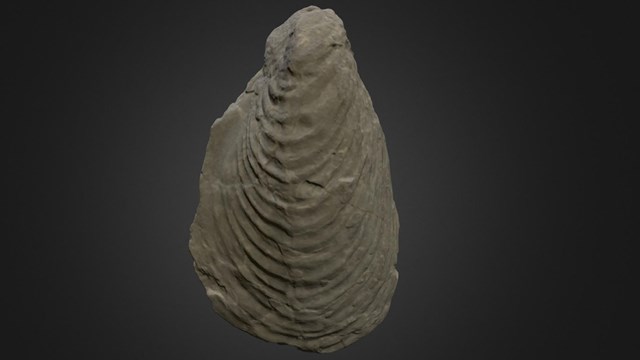The image depicts an elongated, tall, and rippled gray or white rock formation centered against a dark, predominantly black background that lightens at the center. The rock features distinct, wave-like layers or ripples emerging from a smaller top and expanding towards a broader, rounded base, reminiscent of a fossilized object or artifact. The texture suggests petrification, possibly resembling a large petrified shell, a piece of petrified wood, or even a moon rock. The unique ripples and chips along its surface give it an intricate and detailed appearance, with some areas even suggesting anthropomorphic features such as eyes and a mouth, though these are indeed natural formations. The contrast against the dark background draws attention to its textured and layered structure, emphasizing its possible historic or natural significance.